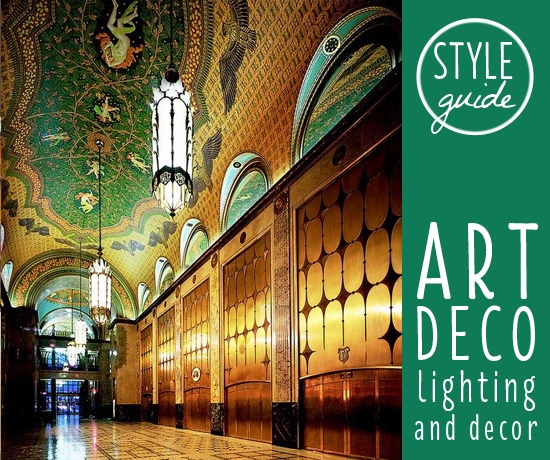The image is a portrait-oriented color photograph showcasing an advertisement for an Art Deco style guide. Dominating the right side of the image is a green vertical bar with white text that reads "Style Guide" inside a white ring, and below, in larger white text, it says "Art Deco" with "Lighting and Decor" in slightly smaller text beneath it. To the left, displaying the grandeur of an Art Deco building's interior, the photograph reveals an opulent hallway. The hallway features large gilded doors and arched niches on the right side, adorned with gold metallic panels patterned with interconnected diamond shapes in dark brown. Below these panels, strips of brown speckled marble adorned with round medallions enhance the luxurious decor, while sections of copper with arching centers add an additional layer of richness. The floors are reflective, basking the space in a golden hue. The ceiling is a masterpiece, domed and decorated with an elaborate Art Deco mural that transitions from a central green area with leaf designs and figures that appear to be sleeping angels, surrounded by eagles, to areas of reddish, white, and finally a predominant yellow hue accented with black designs. Two pendant light fixtures, long and wide, hang from the ceiling, featuring diamond-like shapes and fancy black wrought iron details, emitting white light and adding to the overall dazzling effect of the space.